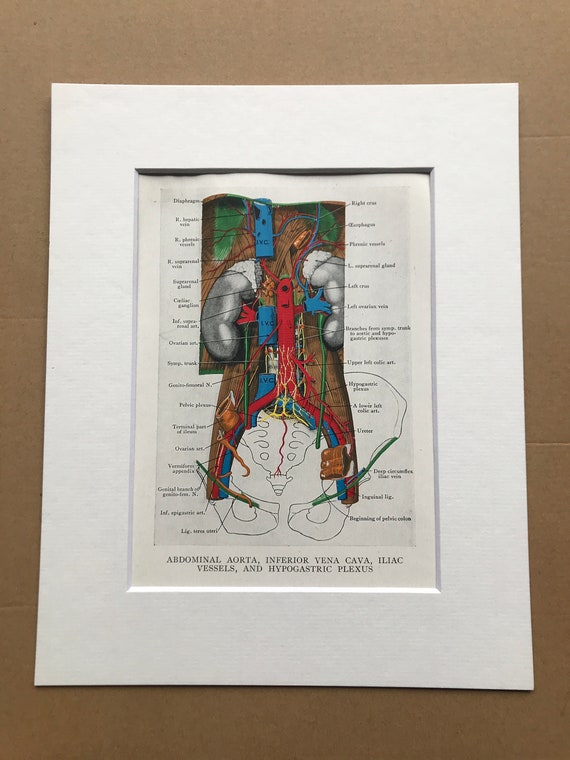This image depicts an anatomical diagram displayed in a white frame mounted on cardboard, though the mounting is slightly wrinkled. At the bottom of the diagram, black text clearly labels key anatomical structures: "abdominal aorta," "inferior vena cava," "iliac vessels," and "hypogastric plexus." The main focus of the illustration appears to be the organs located just above the pelvis, featuring kidneys depicted in gray with one having red and blue veins, possibly indicating arteries and veins or aortas. Central to the image are large red and blue columns showing vascular structures and organs in cutaway views. The drawing, created with pen and marker, includes the pelvic bones portrayed in black lines splaying outward, and the background is filled with various detailed labels pointing to different body parts, though these labels are too small to read clearly at this resolution. The overall color scheme includes subdued shades of gray, brown, red, and blue, giving the parts a somewhat earthy tone.